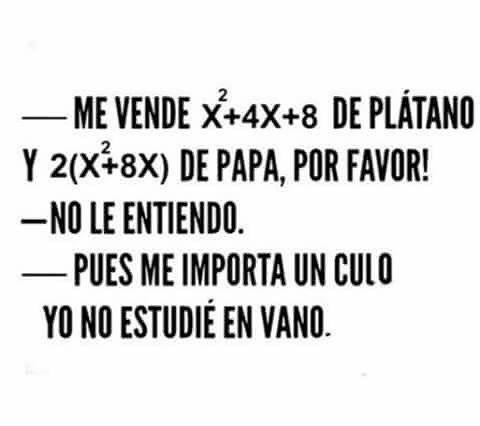The image features a square composition with an all-white background. In the center, starting from about a quarter of the way down, there's a black horizontal line. Below this line, large black text reads "ME VENDE". Following this, there's a math equation: "x^2 + 4x + 8". The next line of text says "DE PLÁTANO", with an asterisk over the "A" in "PLÁTANO". 

Below this, a large "Y" is printed prominently, followed by another math equation in parentheses: "2(x^2 + 8x)" and the words "DE PAPA, POR FAVOR!". The third line contains a horizontal dash, followed by the words "NO LE ENTIENDO." Another horizontal dash is present in the next line along with the text "PUES ME IMPORTA UN CULO." The final line states "YO NO ESTUDIÉ EN VANO."